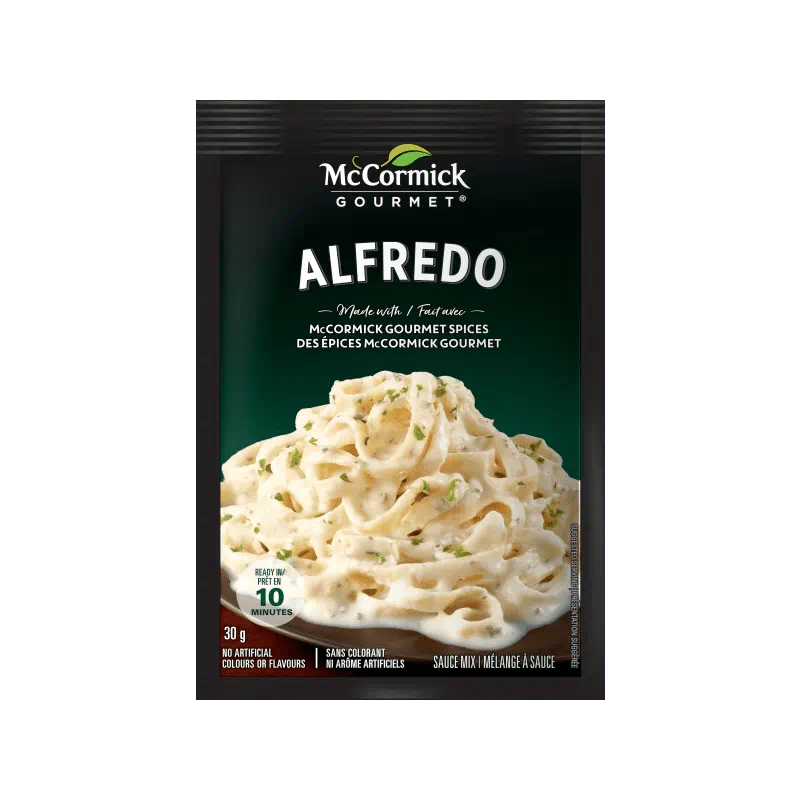The image features a packet of McCormick Gourmet Alfredo Sauce Mix against a white background. The packaging is predominantly dark green, almost black in certain areas. At the top center, the McCormick Gourmet logo is displayed in white text, accompanied by a two-tone green leaf. Below the logo, "Alfredo" is prominently featured in bold, capital letters. The text "made with McCormick Gourmet Spices" appears in a cursive-like font, followed by a translation in French: "Des Épices McCormick Gourmet." The packet shows an inviting image of fettuccine Alfredo, with light cream-colored sauce and sprinkled green herbs. In the bottom left corner, within a circle, it states "ready in 10 minutes," and nearby the packet size is indicated as 30 grams, noting "no artificial colors or flavors."